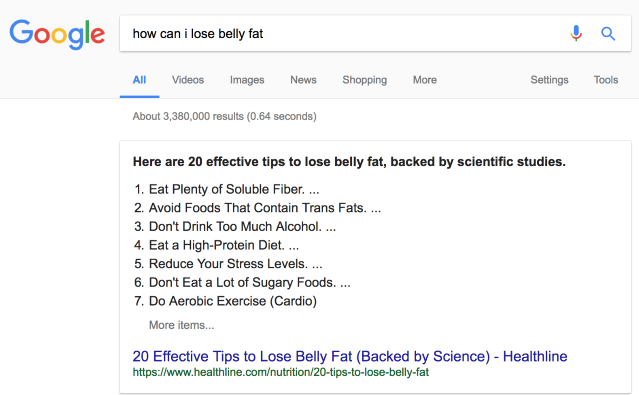The image is a screenshot capturing the results page of a Google search for the query "how can I lose belly fat." At the top, the iconic Google logo is displayed in blue, red, yellow, and green. Below the search bar, you can see microphone and magnifying glass icons in red, gold, and blue, respectively. The search results interface includes a blue "All" tab, followed by gray submenus labeled "Videos," "Images," "News," "Shopping," "More," "Settings," and "Tools." 

A gray line demarcates sections of the page. Immediately below, the number of search results and the search duration, 0.64 seconds, are displayed. The main content begins with a white box bordered by a thin gray line. The box contains black text titled "Here are 20 effective tips to lose belly fat backed by scientific studies," listing seven tips: 

1. Eat plenty of soluble fiber.
2. Avoid foods that contain trans fats.
3. Don't drink too much alcohol.
4. Eat a high protein diet.
5. Reduce your stress levels.
6. Don't eat a lot of sugary foods.
7. Do aerobic exercise (cardio).

A clickable blue hyperlink reading "20 effective tips to lose belly fat backed by science. Healthline." is mentioned, directing to a Healthline article. The URL of the article, displayed in green, is http://www.healthline.com/nutrition/20-tips-to-lose-belly-fat. There are no other notable objects present in the image.